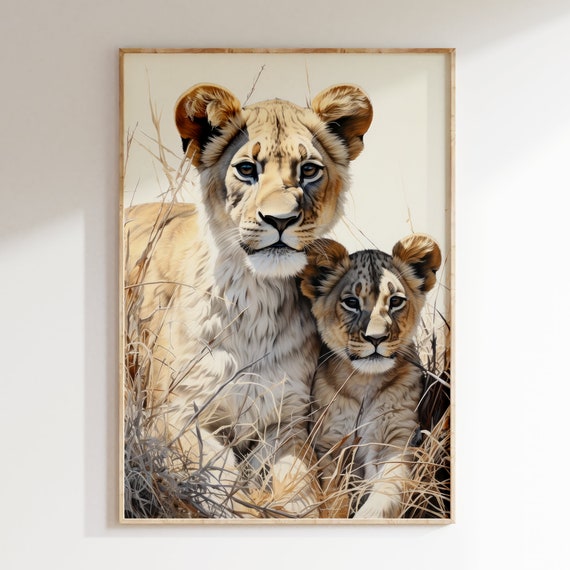The detailed photograph showcases a poster of artwork depicting a serene and intimate scene of a lioness and her cub. The overall shape of the image is square, with the photograph centered within a light brown wooden frame hanging on a white painted wall. The rectangular poster within the frame has sides twice as long as its top and bottom edges. The artwork captures a majestic adult lioness with a golden brown back and head, and white fur adorning its chest, neck, lower mouth, and stomach, laying down on the grass. To her right rests a similarly colored cub, mirroring her graceful repose. Both lions are poised on what appears to be a grassy terrain, with brownish, dried blades of grass interspersed with hints of green visible at the bottom left and right sides of the poster. Their keen eyes look directly at the camera, adding a captivating and lifelike essence to the painting.